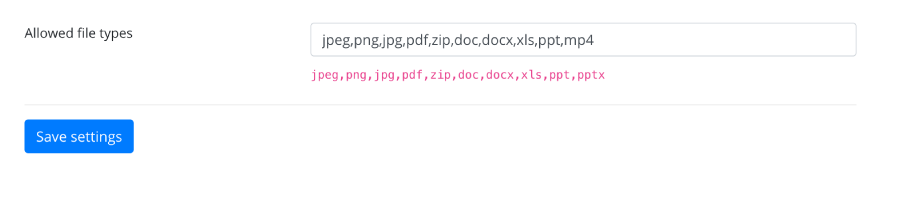The image depicts a user interface for managing allowed file types within a rectangular input box. Inside this box, the user has specified a list of permitted file extensions, including: jpeg, png, jpg, pdf, zip, doc, docx, xls, ppt, and mp4. To the left of this box is the label "Allowed File Types," indicating the purpose of the input box.

Directly beneath this box, a series of default allowed file types appears in red text, displaying the extensions: jpeg, png, jpg, pdf, zip, doc, docx, xls, ppt, and pptx. Noteworthy is that the red-highlighted list matches the user's input except for the inclusion of "pptx" instead of "mp4" in the user's list.

Additionally, a blue "Save Settings" button is positioned in the bottom left corner of the interface, suggesting that users can save any modifications to the list of allowed file types by clicking this button. This interface appears to enable users to customize file type permissions, possibly overriding defaults with new settings.